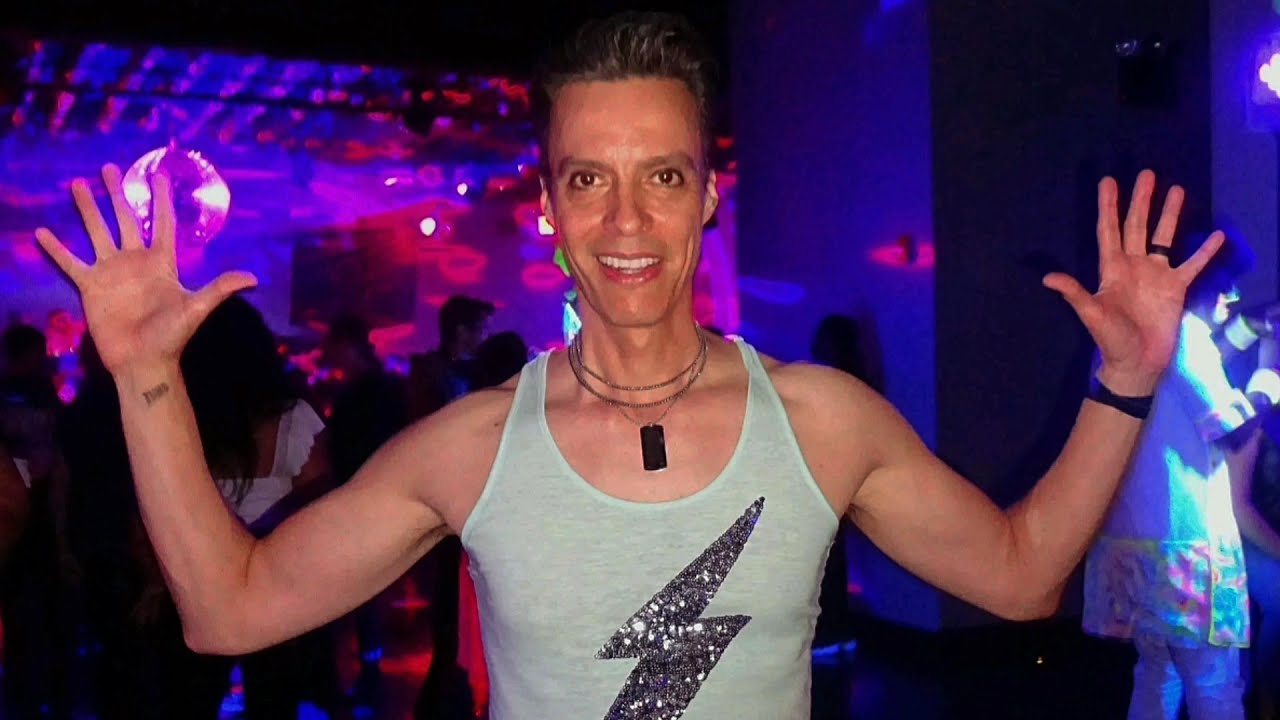The photograph captures a man at what appears to be a nightclub, illuminated by vibrant neon blue, purple, and pink lights. He is smiling directly at the camera with his arms raised, elbows bent, and fingers spread wide, giving a playful and energetic vibe. The man is light-skinned with dark eyes, short sides and poofy hair on top, and a joyful expression showcasing his white teeth. He is adorned with several necklaces, including a distinctive dog collar-like one, and dons a light gray tank top featuring a glittery, sequin lightning bolt cutting through the center. His left hand sports a black bracelet and a black wedding band, while his inner right wrist is marked with a small tattoo. In the hazy background, the nightclub’s dynamic atmosphere is evident with people milling about under the colorful lights, enhancing the lively and festive setting.